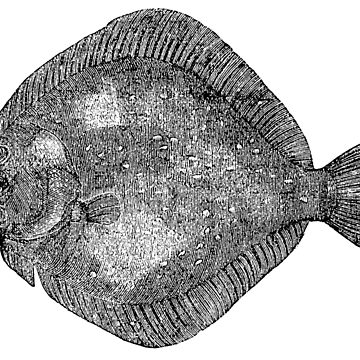The image depicts a black and white side view of a fish fossil, set against a white background, facing left. The fossil appears almost transparent, with detailed features that have aged and weathered over time. The head and snout on the left side are cut off, as well as the end of the tail on the right. Prominent features include a visible eye on the left, various gills leading towards the center, and fins positioned on the top, bottom, and sides of the body. The fish's scales are most noticeable in strips along the top and bottom edges, as well as on the distinct tail. The entire fossil is speckled with numerous white spots, adding to its ancient and potentially indigenous appearance.